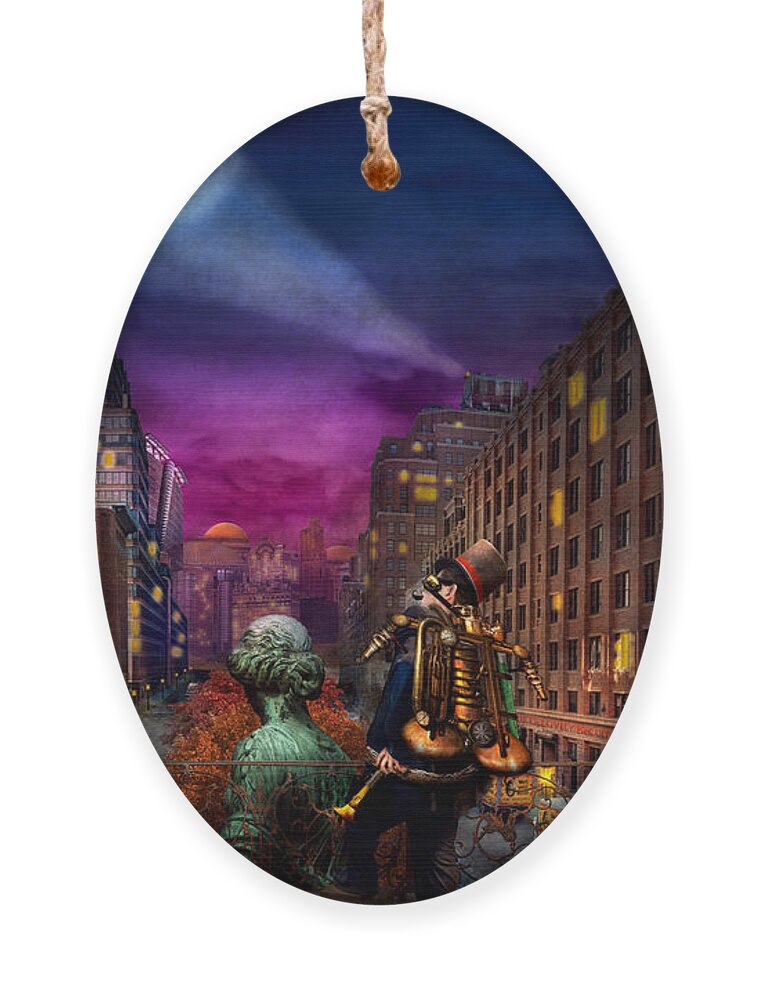This is an oval, digitally created painting that appears to be intended to hang from light-colored twine tied through a circular notch at the top, almost like a pendant. The image depicts a cityscape at night, with a spotlight piercing a bruised purple-pink sky adorned with misty, purple clouds. Below the colorful sky, an orange dome suggests a setting sun.

Prominent tall buildings rise on the right side of the street, contrasted by shorter buildings on the left. Illuminated yellow windows highlight the scene, although many remain dark, emphasizing the night-time setting. Down the center of the wide street, brown leafless trees stand, perhaps indicating a fall or winter season, while a diffuse crowd of circled heads lines up down the street.

In the foreground, there are two notable figures with their backs to us. On the left stands a statue of a woman, seemingly made of aged bronze with a green patina. Her hair is styled up in a French knot. To the right, a man wearing a blue jacket, blue pants, and a brown and red top hat carries a peculiar assortment of steampunk brass musical instruments on his back. He holds a horn-like device in his left hand, and his positioning creates an intriguing optical illusion, making it unclear if he is enormous or floating. The entire composition is rendered predominantly in shades of browns, purples, and blues, lending a dreamlike, surreal quality to the artwork.